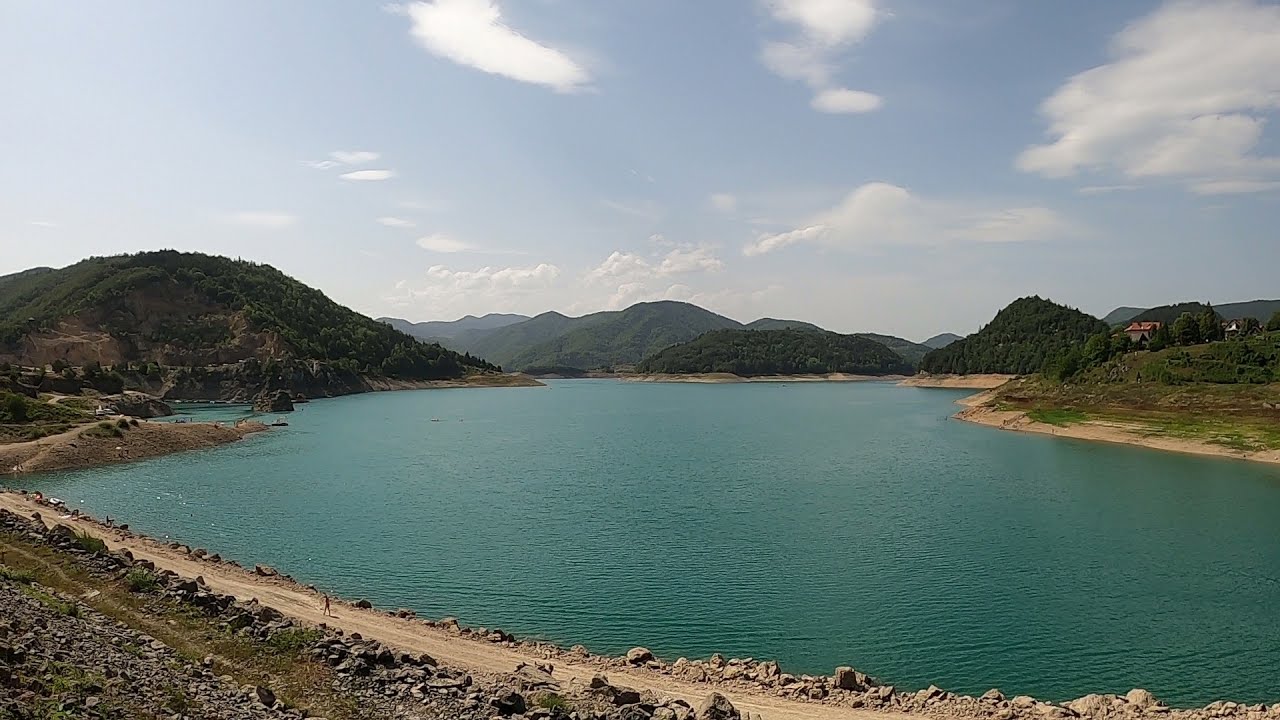This image captures a stunning landscape featuring a large, serene lake or reservoir surrounded by rolling hills and distant low-hanging mountains. The turquoise water is calm and flat, reflecting the fluffy white clouds scattered across the grayish-blue sky. The scene appears to be set on a sunny day, possibly in the early afternoon, allowing for clear visibility of the rich greenery enveloping the landscape. A dirt path edged with rocks and boulders runs diagonally in the foreground, where a lone person can be seen running. This path is flanked by lush grass, bushes, and trees, adding to the rural charm of the area. In the distant background to the right, a house with distinctive red, stucco-type roof tiles peeks out, adding a touch of human presence to the otherwise natural setting. The horizon is roughly in the middle of the image, accentuating the vast expanse of the turquoise lake and the undulating hills that fade into the distance.